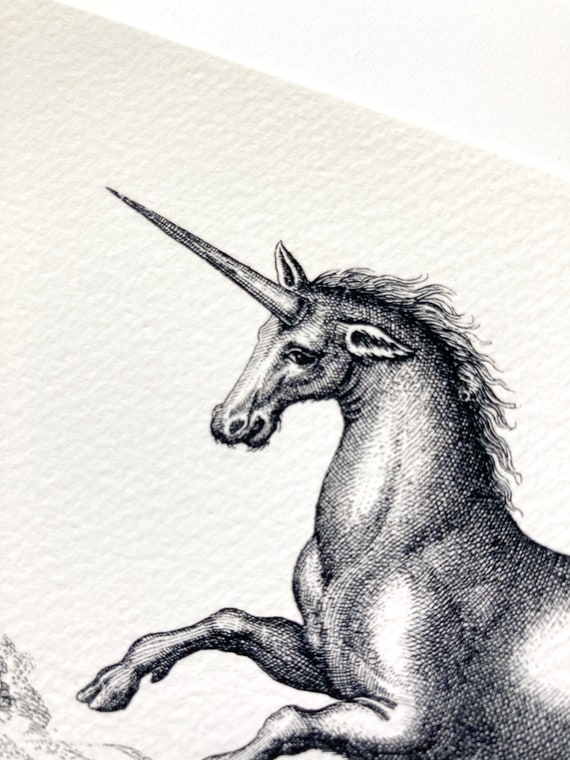This image showcases an angled view of a meticulously detailed pencil drawing of a unicorn, rendered in black and gray tones on thick, textured white drawing paper laid against a white surface. The sketch captures only the top half of the unicorn, emphasizing its muscular build and robust, thick neck, which appears almost too large for its relatively small head. The unicorn's long, straight, conical horn is prominently featured atop its head. The intricate texture of the lines on its body resembles a fingerprint pattern, adding depth to the depiction. Fine hairs are illustrated on its chin and underneath its face, enhancing its lifelike quality. The background of the image ranges from cream-colored to textured cream, with a subtle hint of a hillside or mountain in the bottom left corner. The unicorn’s ear position adds a quirky aspect to its appearance, and its hooves, slightly atypical for a horse, further contribute to its unique, fantastical nature.